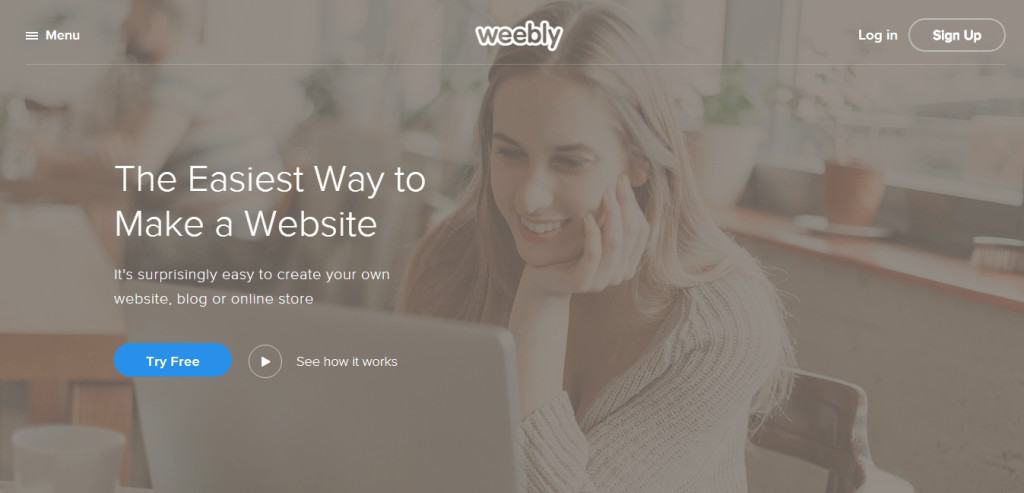This horizontal screenshot captures the homepage of the Weebly website. At the top center, the Weebly name is prominently displayed. A menu button is located at the upper left corner, while the login and sign-up buttons are positioned at the upper right corner. 

Bold, white text to the left of the center reads, "The easiest way to make a website," with a subtitle in smaller text beneath it that says, "It's surprisingly easy to create your own website, blog, or online store." Below this, an oval blue button prompts users to "Try Free." Adjacent to this button is a circular play button with a triangle icon, accompanied by the text, "See how it works."

The rest of the webpage is overlaid with a translucent gray, revealing a background photograph. In the image, a woman with long blonde hair is seated at either a laptop or desktop computer. She is wearing a ribbed sweater, smiling, and resting her face on her hand with her elbow on the table. To her right, plants adorn a windowsill, contributing to a cozy atmosphere. To her left, there is a desk or some other surface, and the shadow of another person, likely a man, is visible, looking off towards the upper left corner of the image. The overall scene conveys a sense of focus and engagement in a comfortable and productive setting.